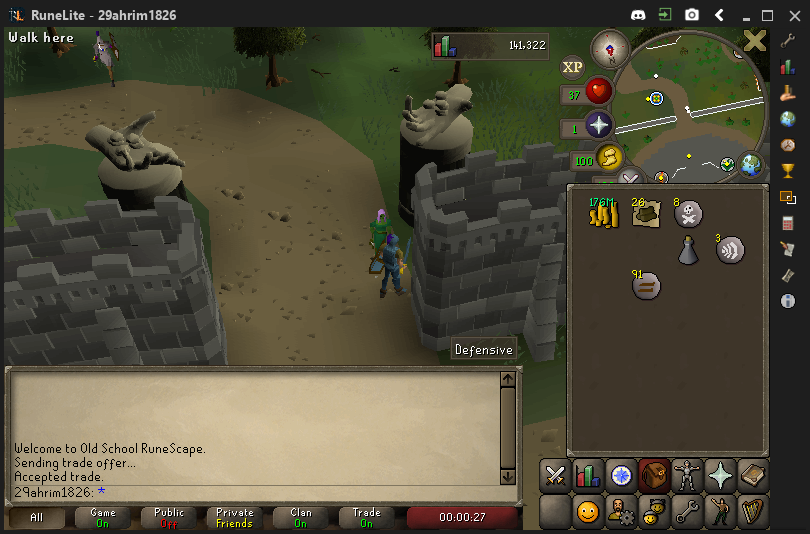This is a detailed screenshot from the game RuneScape, specifically using the RuneLite client. The top left corner features the text "RuneLite" along with numerical data, possibly referring to a username or session ID. Dominating the center of the image is the main game view, showing a character exiting a castle and heading towards a wooded area. The castle is surrounded by high walls, with colors predominantly in shades of brown, green, and beige. 

In the bottom left of the screen, there's a chat interface where players can communicate, with visible messages such as "Welcome to Old School RuneScape," "Sending Trade Offer," and "Accepted Trade." The right hand side of the screen is filled with graphical user interface elements, including multiple icons and rectangular buttons that display various in-game stats and counts. A round map orients the player, located in the upper right-hand corner, complete with a compass and a "big X." According to the GUI, the player possesses 176 million coins. There's also a mention of the username "a h r i m 1826." 

In summary, the image meticulously captures both the navigational elements and the interactive features of the RuneScape game interface, highlighting the player’s position, chat functionality, and statistics.